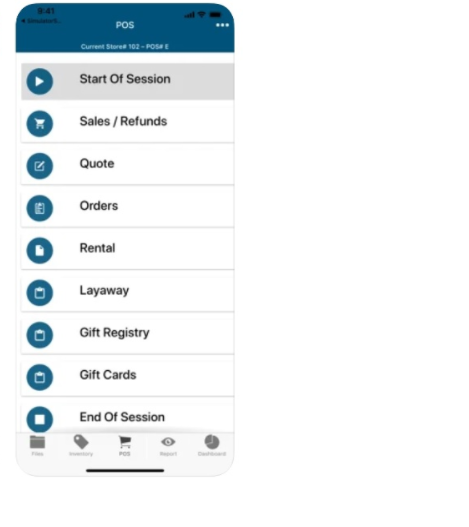The image features a white background with the PLS logo prominently displayed at the top. The digital clock reads "9:41", indicating the current time. Below, the current store number is identified as "#102" along with additional alphanumeric codes. 

A gray rectangle marks the "Start of Session" button, accompanied by various operational options including "Sales/Refunds", "Quote Orders", "Rental", "Layaway", "Gift Registry", "Gift Cards", and "End of Session". 

At the very bottom, another gray rectangle houses several icons: "Files" represented by a document folder, "Inventory" depicted with a sales tag, "POS" shown with a shopping cart, "Report" symbolized by an eye, and "Dashboard" illustrated with a pie chart. The center of the bottom section features a noticeable black bar.